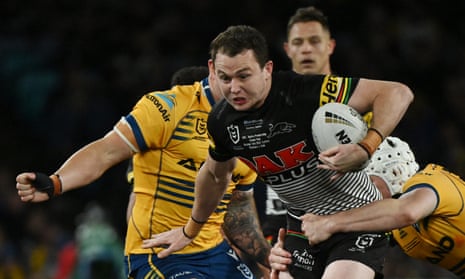In the midst of an intense rugby match, a player wearing a black jersey adorned with red and white accents and black shorts is at the center of the action. The black jersey features the letters "A" and "K" in red, with "P plus" in white below, and black and white stripes at the bottom. On the right shoulder, a yellow bar reads "HER." The player with black hair clutches the white rugby ball tightly while getting tackled around the waist by an opponent in a yellow jersey and a white helmet. The yellow team's jerseys have blue accents and they wear blue shorts. Another player in a yellow jersey and blue shorts, his shirt featuring a logo and partial text ending in "NAI," is sprinting towards the skirmish from the left. In the background, another yellow jersey player stands with his mouth slightly open, observing the heated clash. The scene is set on a rugby field, showcasing the dramatic intensity of the sport.